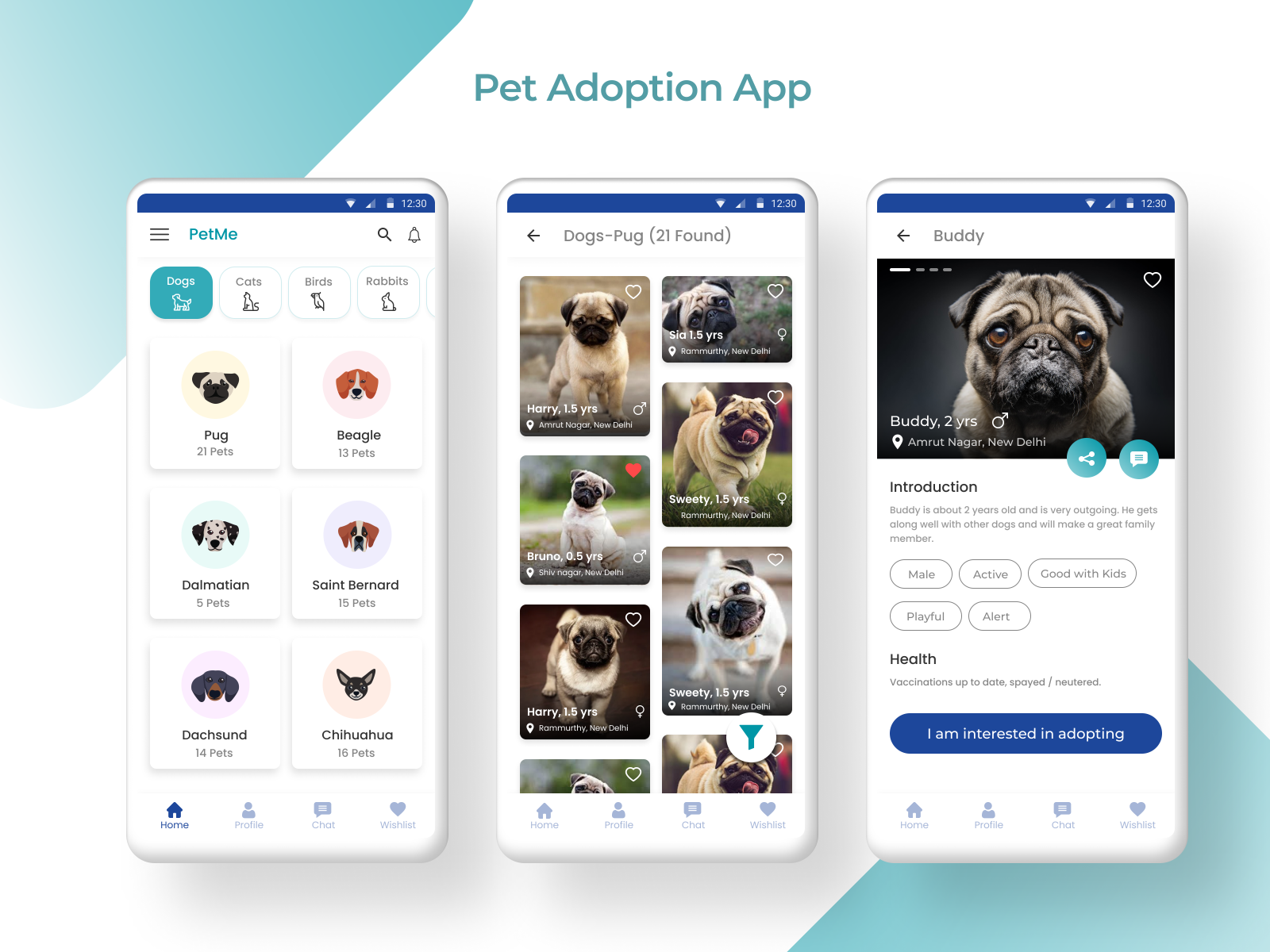The image is of a pet adoption website featuring a clean, white background. The design includes light green accents in the upper left and bottom right corners. Prominently displayed at the top is a green label reading "Pet Adoption App."

In the center of the image are three white cell phones, each displaying different screens of the app. The first phone screen showcases the app’s main menu. At the top, a green header reads "Pet Me." Below this, there are tabs for various types of pets: Dogs, Cats, Birds, and Rabbits, with the 'Dogs' tab highlighted. Various dog breeds are listed under this tab with the number of available pets for each breed: Pug (21 pets), Beagle (13 pets), Dalmatian (5 pets), St. Bernard (15 pets), Dachshunds (14 pets), and Chihuahuas (16 pets).

The second phone screen shows search results for dogs, specifically 21 found, displaying pictures and brief details for each. The pets listed include:
- Harry, 1.4 years
- Sia, 1.5 years
- Bruno, 0.5 years
- Sweetie, 1.5 years
- Harry, 1.5 years
- Sweetie, 1.5 years

There is also a filter symbol indicating the user can refine their search.

The third phone screen is dedicated to a specific dog named Buddy, showcasing a detailed profile:
- Buddy, 2 years old, male
- Located in Amrut Nagar, New Delhi
- Description: "Buddy is about 2 years old and very outgoing. He gets along well with other dogs and will make a great family member."
- Traits: Male, active, good with kids, playful, alert, healthy
- Health: Vaccinations are up to date, spayed/neutered

At the bottom, there is a blue button labeled "I'm interested in adopting." This call-to-action allows users to express their interest in adopting Buddy.